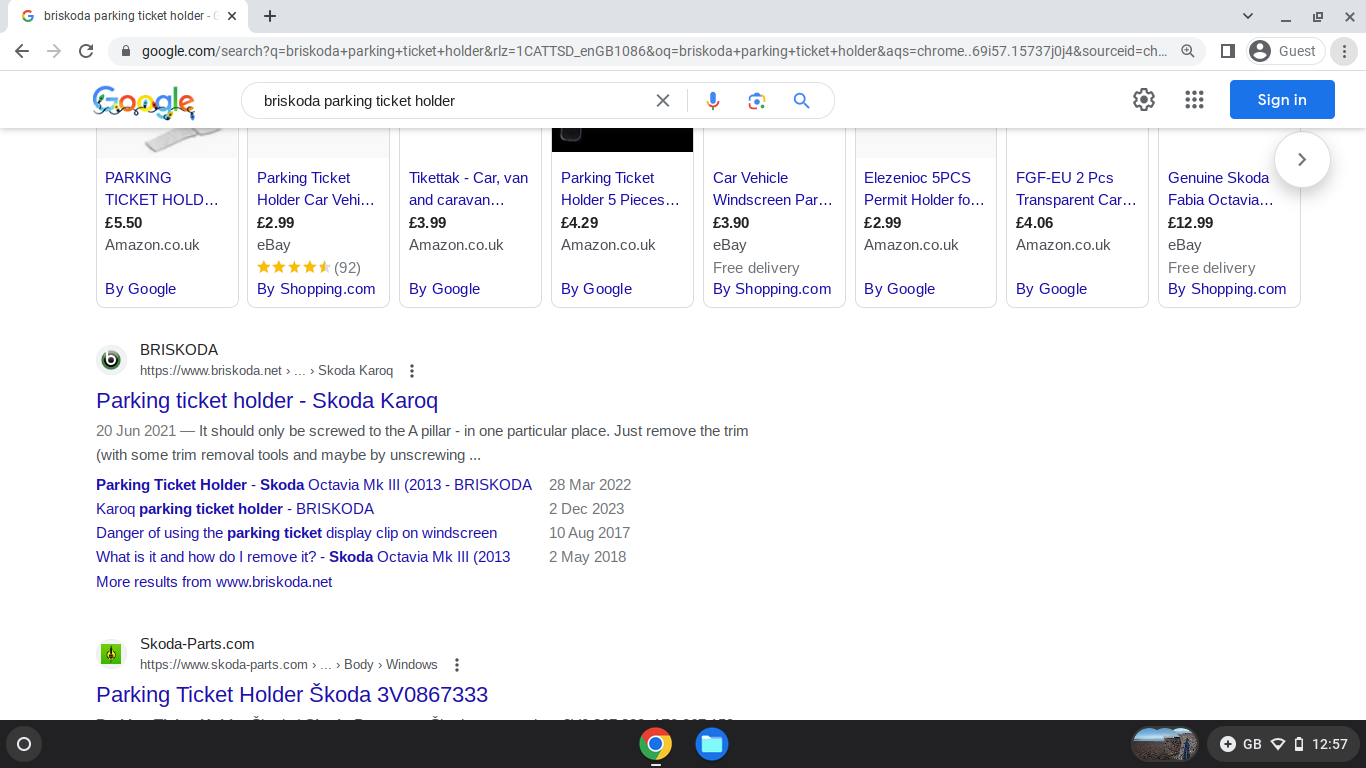The image is a screenshot from a computer displaying the results of a Google search for "Briscota parking ticket holder." At the top, the search query is seen in the search box, adjacent to the Google logo, which is decorated with intertwined Christmas lights. Below the search bar, the screen is divided into eight sections, each with a white background and primarily blue and purple text.

1. The first search result states, "Parking ticket hold... £5.50 Amazon.co.uk."
2. The second result similarly lists, "Parking ticket holder, 5 pieces, £4.29 Amazon.co.uk."

There are a total of eight such results displayed across the screen. Further down the page, a result features a circle with a 'B' in it, next to the description "Briscota parking ticket holder SCOTACAROQUE," followed by additional text, including references to "SCOTA OCTAVIA MK3."

Another notable search result is marked by a blue square with a symbol, reading "SCOTAPARTS.COM parking ticket holder SCOTA."

At the bottom of the screenshot, there is a long black bar, likely the browser's taskbar, containing various icons including the Google Chrome logo and a blue circle with a flag-like symbol.